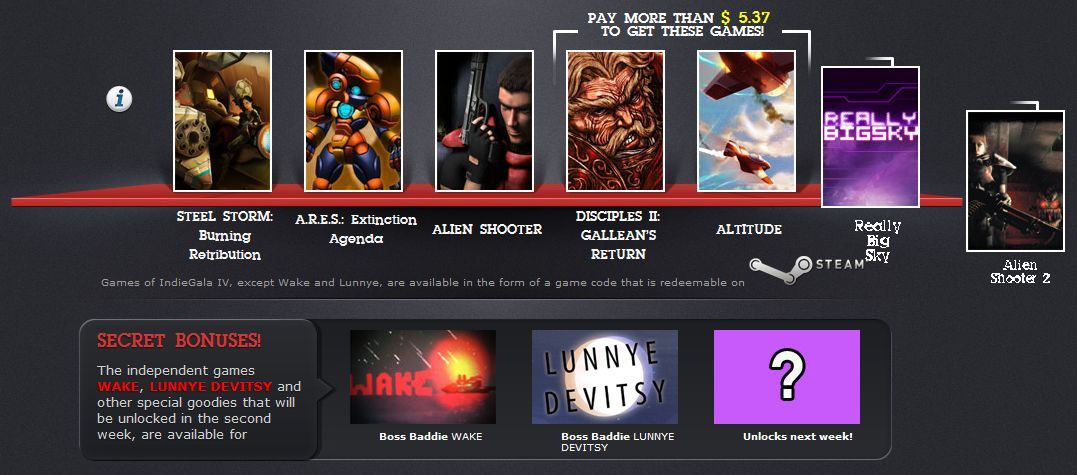The image is a black, horizontally oriented rectangle featuring a row of seven game covers. The covers are arranged side by side, but the last two are staggered vertically. 

From left to right, the games are:
1. "Steel Storm: Burning Retribution"
2. "A.R.E.S.: Extinction Agenda"
3. "Alien Shooter"
4. "Disciples II"
5. "Galleons Return"
6. "Altitude" 
7. "Really Big Sky" (positioned slightly lower)
8. "Alien Shooter 2" (positioned even lower).

Between "Disciples II" and "Altitude," there is a bracket enclosing the game covers, with a message above it stating, "Pay more than $5.37 to get these games," where "Pay more than" and "to get these games" are in white text, and "$5.37" is highlighted in yellow.

Below the game covers, there is an additional message in white text stating, "Games of Indie Gala 4 except Wake and Lunenye are available in the form of a game code that is redeemable on Steam."

Another line below this mentions additional content: "Secret bonus: The independent games Wake, Lunenye, Devisty, and other special goodies that will be unlocked in the second week are available." The word "Devisty" is spelled out as "D-E-V-I-S-T-Y."